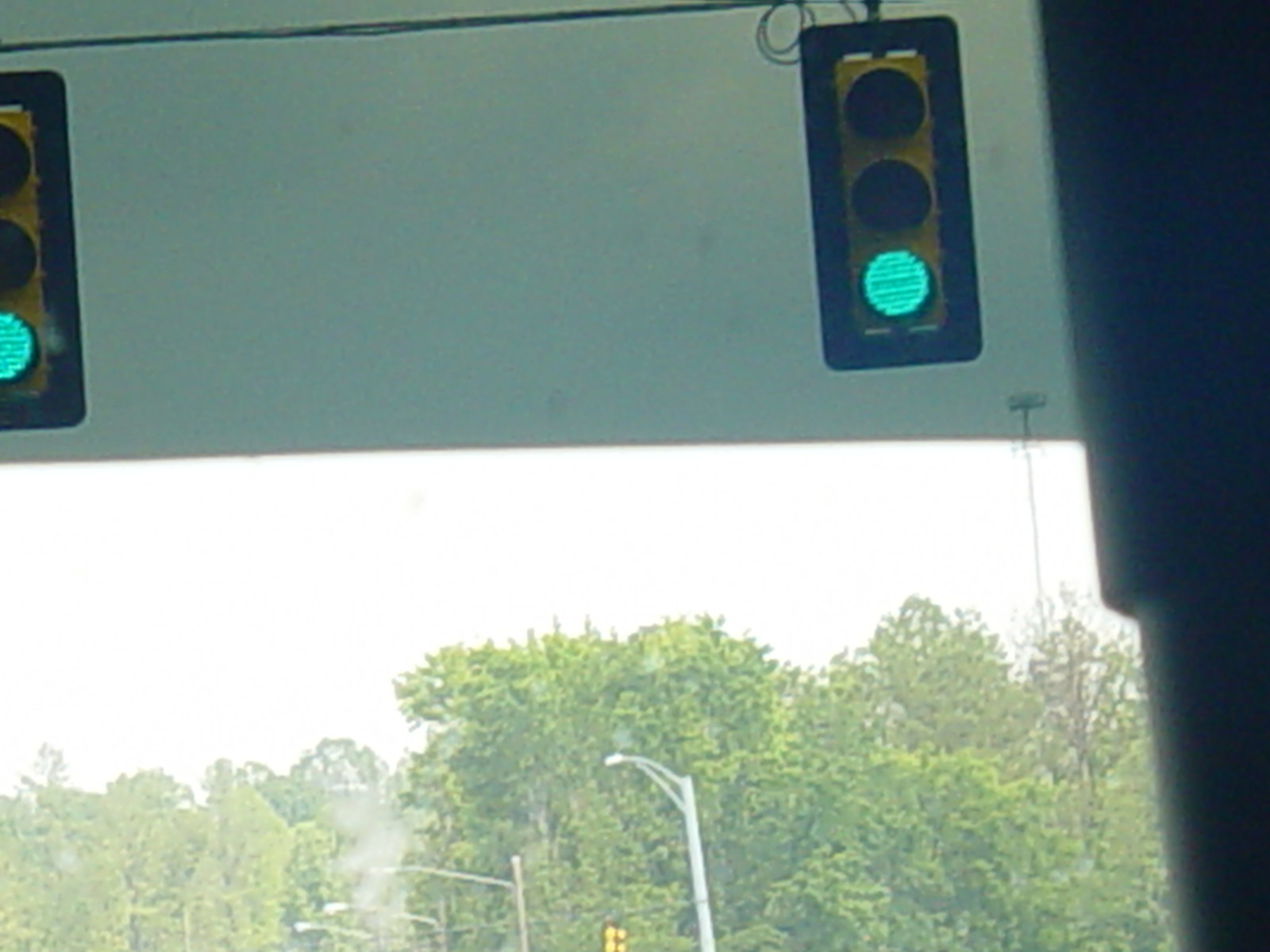The photograph appears to be taken from inside a car, looking out through a partially tinted windshield, which shades the upper section of the image. At the top, two vertically-oriented, rectangular traffic lights with yellow casings and black outlines can be seen, both displaying illuminated green lights with horizontal lines. The leftmost traffic light is partially cut off. These traffic lights are suspended from wires, with some curling visible on the wire above the right traffic light. Below the traffic lights, there are at least four tall, gray street lamps, spaced about five feet apart. The bottom half of the image features a clear, partly cloudy sky with numerous tall, green trees. Additionally, the photograph shows the top of another traffic light below the rightmost pole and a black pole on the right-hand side, which partially obscures the view. The scene outside appears to be bright and the overall setting gives off a sense of being taken at an intersection while the car is stopped.